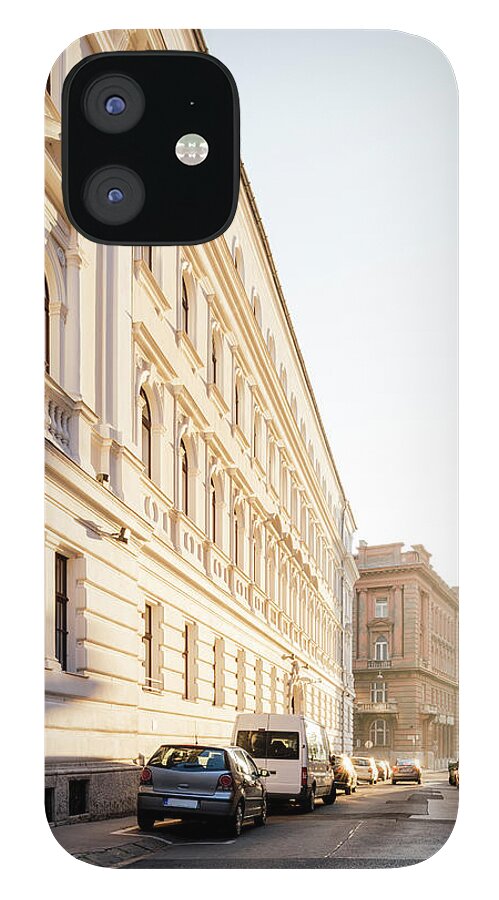This image depicts the back of an iPhone case, featuring an intricately detailed street scene. The case is designed with a photograph of a bustling street on an overcast day, portraying classic, urban architecture. Dominating the scene is a tall, creamy white four-story building with elegant curved and carved windows and fine brick and woodwork, situated from the upper left to the lower left corner of the image. Adjacent to it, a beige building adds depth to the background.

In the lower center of the image, a street populated with several parked cars extends into the distance. On the left side of the street, there are multiple cars parked, including a van and an SUV, with parking spaces extending onto the sidewalk. On the right side, a single car is driving down the road and another car is visible further in the distance. The sky above the scene is light blue, reflecting the overcast weather. Enhancing the realism, the iPhone's triple camera setup is prominent in the upper left corner of the case, capturing this vivid urban tableau.